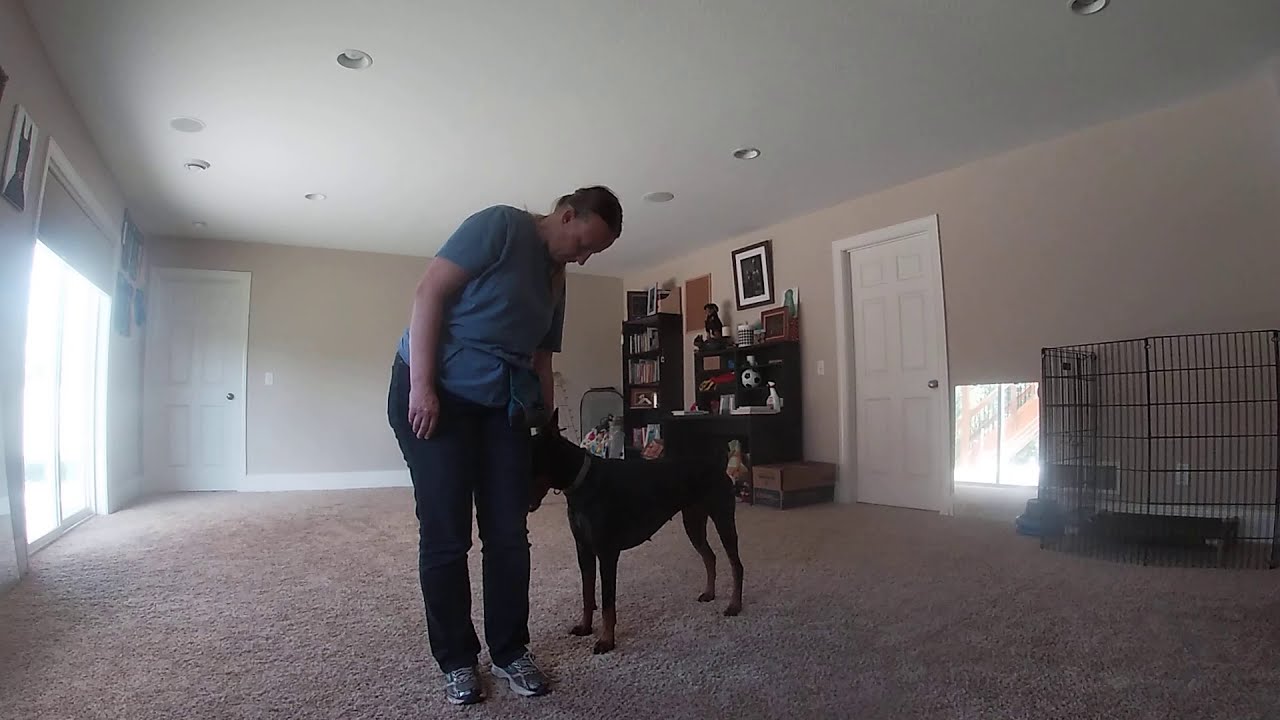The photograph depicts a large, sparsely furnished living room inside a house. The room features beige walls, a white ceiling with spotlights, and light brown carpet. In the center stands a person dressed in dark jeans, sneakers, and a short-sleeved blue shirt, with short brown hair. They are leaning over to pet a large black dog, which appears to be a Doberman with pointy ears and a red collar. The person’s gesture suggests a moment of affection as they interact with their pet. 

In the background, there are a couple of white doors with bronze handles and some windows on the far left allowing bright daylight to stream in. The scene includes minimal furnishing, consisting of a black dog crate positioned against the far right wall, a bookcase filled with books, and a table cluttered with various items. Despite the large, open space, the room feels cozy and intimate, primarily designed for comfortable interaction between the person and their dog.